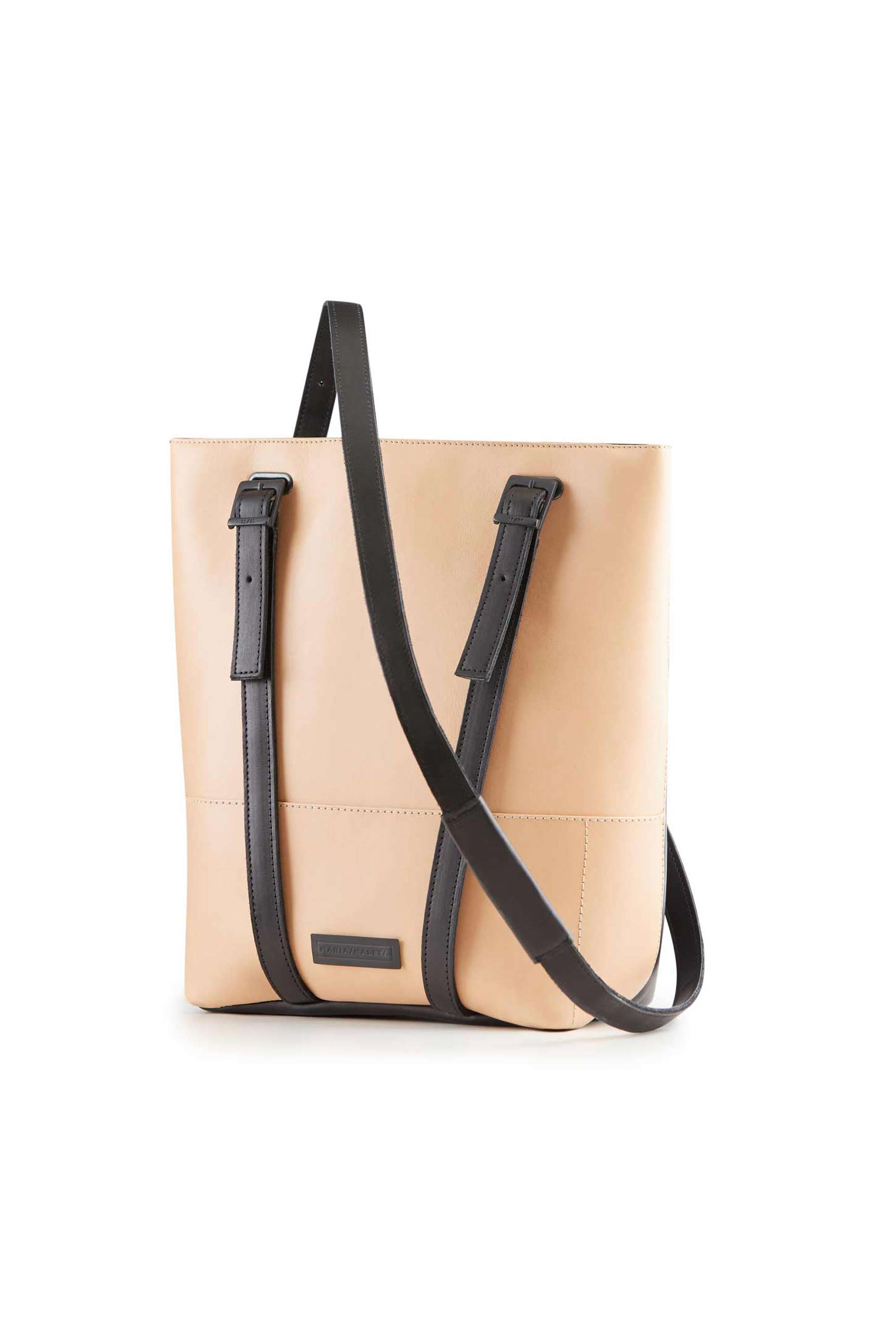This is a photograph of a stylish and multifunctional tote backpack crafted from high-quality taupe beige leather by Maria Moletta. The bag features a blend of elegant and durable design elements, making it both functional and visually appealing. Notable details include intricate vertical stitching along the midsection and an additional dark brown leather layer at the base to provide extra strength and protect the main compartment. The backpack offers versatile carrying options with its deep brown adjustable leather straps, which resemble belts fastened with actual buckle closures, allowing it to be worn over the shoulder or on the back. A distinctive Maria Moletta emblem adorns the bottom of the bag, adding a touch of brand sophistication. The light beige tones of the leather are accented by the darker brown straps, creating a beautiful contrast that enhances the bag's overall aesthetic. In the background, a faint orange square and some metal structures are visible, providing a subtle context to the elegantly photographed accessory.